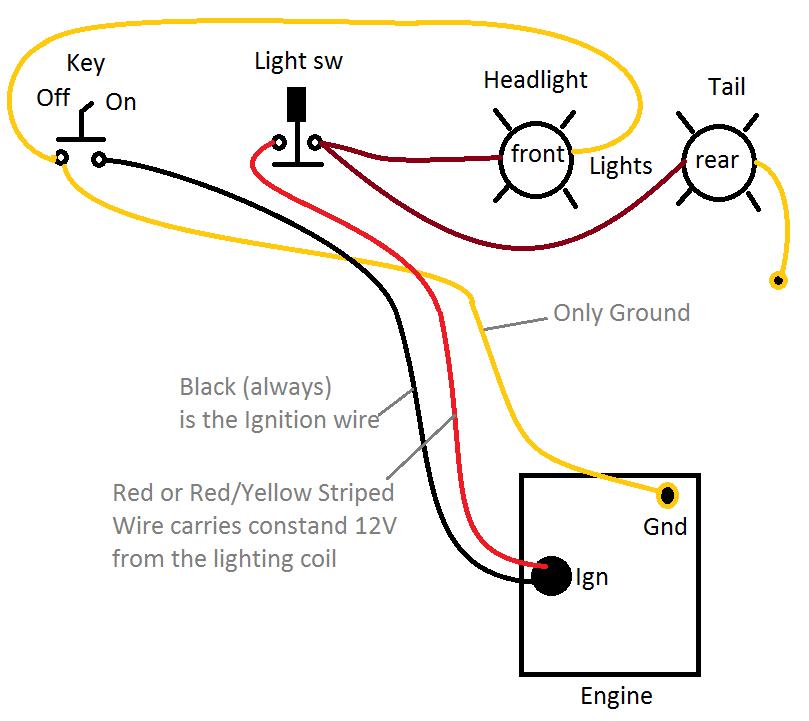The image is a detailed wiring diagram on a white background without visible borders. The diagram displays connections from various components, notably focusing on key switches, light switches, and headlights. At the top left, a label marked "key" indicates two positions: "off" and "on," with associated wiring—including a black wire to the "on" position and a yellow wire to the "off" position. Adjacent to this is the "light SW" section, illustrated as a lamp stand with two circles beneath it. A red wire connects to the left circle, and two maroon wires emerge from the right circle heading towards other parts of the diagram.

To the right, there's a central circle labeled "headlight." The inner label reads "front," and connected to this circle are wires from various sources, including a maroon wire from the light switch and another yellow wire from the key switch. Additionally, aligned to the right of the headlight circle, there's another circle marked "rear" with "tail" above it, suggesting a connection to the rear lights. Another maroon wire from the light switch connects here, with a yellow wire extending from this circle.

Descending from these components, multicolored wires (yellow, red, brown, and black) lead downwards to a square box located in the lower right-hand corner. This box is outlined in black, within it a larger circle labeled "IGN" (ignition) and a smaller circle labeled "GND" (ground). The yellow wire labeled "only ground" extends to the smaller GND circle. The black wire, marked as "black (always)" and identified as the ignition wire, and the red wire labeled "red/yellow stripe wire" (carrying constant 12V from the lighting coil) exit from the larger ignition circle.

This diagram effectively represents the wiring layout for an engine, detailing how wires connect from the ignition and various lights to other key components, ensuring correct pathways for electrical currents.